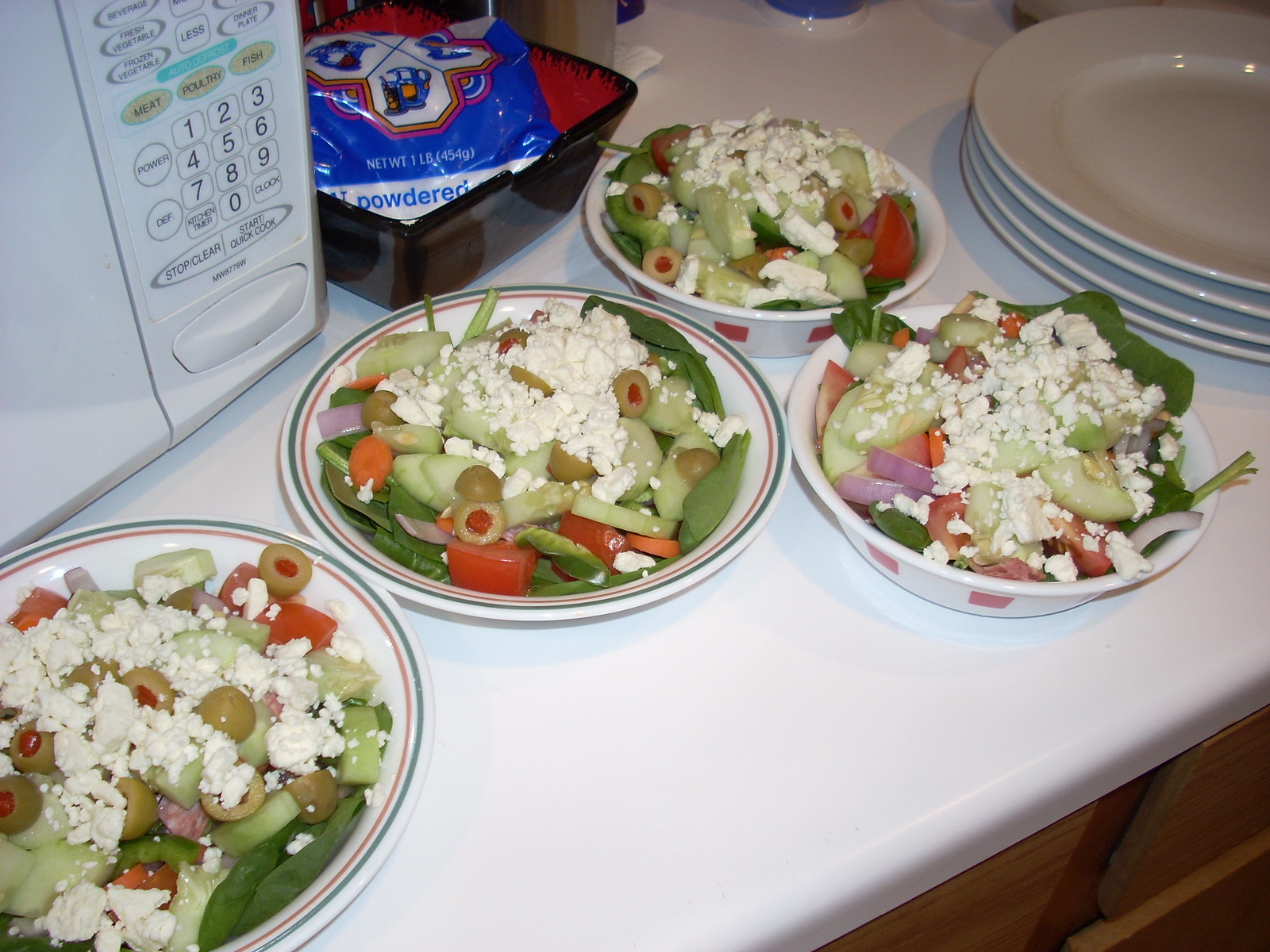On a sleek white countertop rests four generously filled white porcelain salad bowls, each adorned with red and green stripes around their edges. The vibrant salads within feature a base of fresh spinach leaves and cucumbers, topped with juicy tomatoes, sliced green olives, and a generous sprinkle of crumbly feta cheese. Diced onions add to the array of colors and textures, making these salads visually appealing and inviting.

To the left of the salads is a white microwave, its white buttons marked with black text, partially visible alongside a dark brown bowl with a red interior. This bowl cradles a blue plastic bag of powdered sugar. Above the salads, a neat stack of white plates stands ready for use.

The scene combines functionality and visual appeal, set against the contrasting backdrop of brown wooden cabinets and drawers below. The white countertop holds all these elements together, framing a snapshot of a vibrant and organized kitchen space.